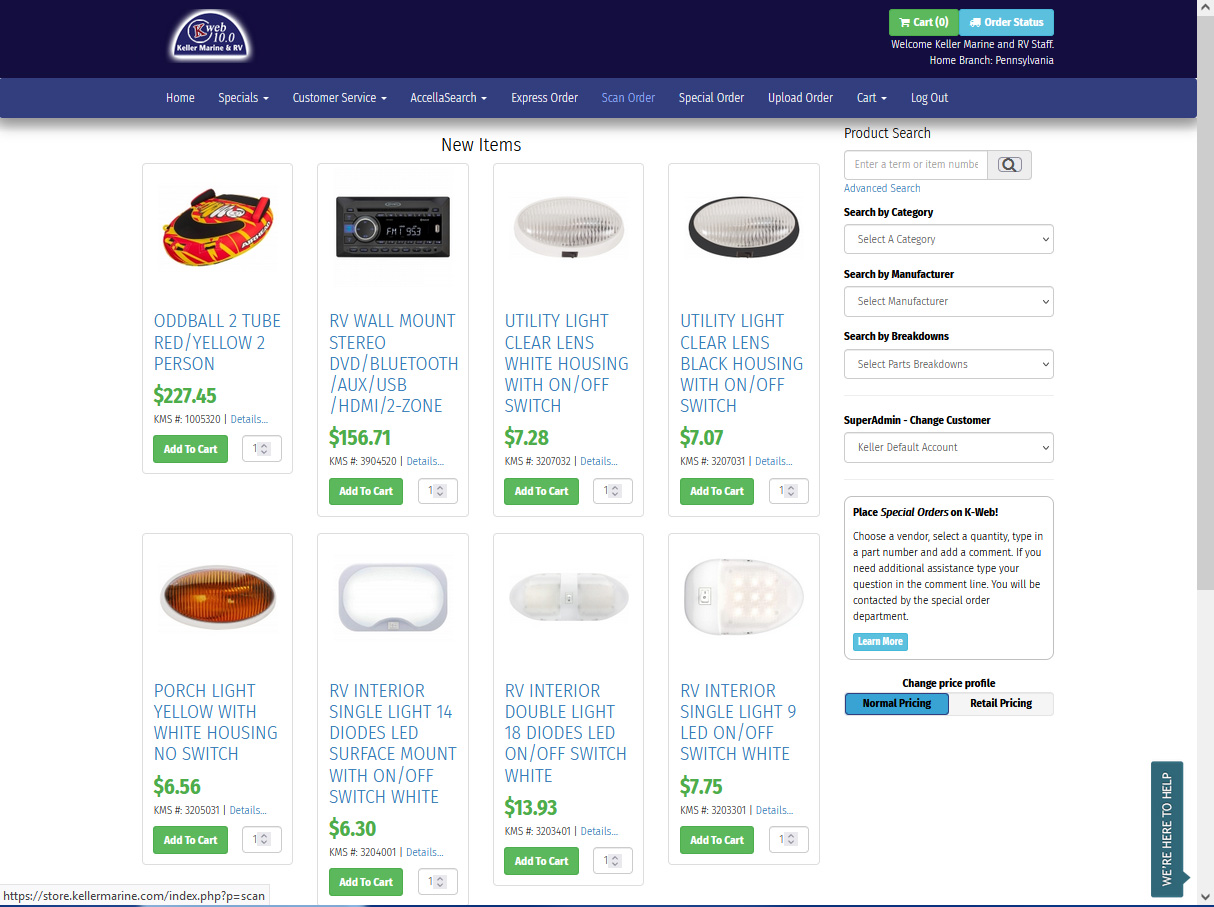The image depicts a webpage with a sleek dark blue border at the top. On the top left corner of this border is the website’s logo. On the top right corner, there's a green cart button for shopping, as well as a blue button labeled "Order Status." Below this blue button, there's a delicate, lighter-colored horizontal line. Underneath this, there is a blurred menu bar, which despite zooming in remains difficult to read. The menu options, from left to right, appear to be: Home, Special, Customer Service, Express Order, Scan Order, Special Order, Upload Order, Cart, and Log Out.

Beneath the menu bar, there is a section labeled "New Items," showcasing eight different product listings in a grid format. Each product is housed within its own box. Starting from the top left:

1. "Oddball Tube, Red, Yellow, Two-person - $229.45"
2. Directly to the right of it: "KB Wall Mount, Stereo, DVD, Bluetooth, Auxiliary, USB, HDMI, Seven Zone - $156.71"

These listings provide a brief description of the items along with their prices, aimed at aiding the user’s shopping decisions.